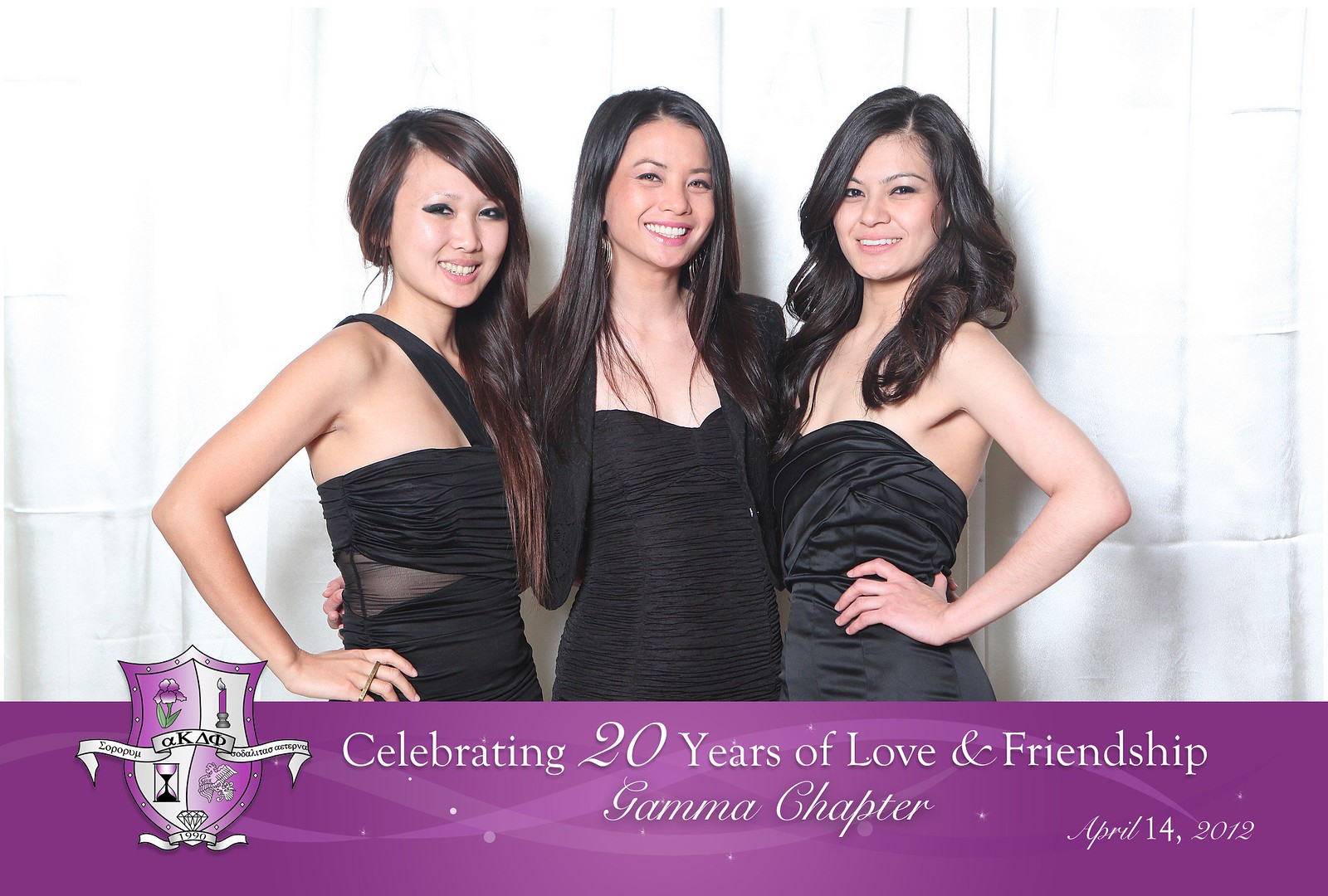This is a color photograph featuring three women standing against a white backdrop. All three women are wearing black dresses, with the woman on the left and the woman on the right both having their right hands on their hips. The woman in the center has her arms behind the two beside her. They are all smiling and appear to be of Asian descent. The woman on the right has brown hair, while the other two have black hair.

At the bottom of the image, a purple band spans the width of the photograph. On the left side of the band, there is a coat of arms or logo that appears to be a shield with a ribbon and is divided into four sections. Next to the logo, in yellow and white text, the band reads: "Celebrating 20 years of love and friendship, Gamma Chapter." On the bottom right of this band, the date "April 14, 2012" is written in white text.